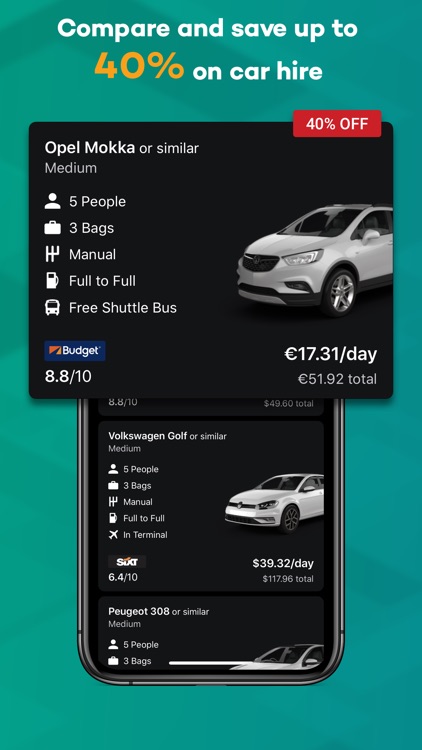Discover unbeatable savings of up to 40% on car rentals! The image features a promotional banner with a blue background and highlights the Opal Mocha as a similar medium option. Showcased are various rental vehicles, including a gray car and a white car, all with competitive pricing and specifications.

One featured offer is the Volkswagen Golf (or a similar medium vehicle), accommodating up to five people and three bags, available for 17.31 EUR per day (15.92 EUR total), with a manual transmission and a full-to-full fuel policy. A budget-friendly choice rated 8.8, perfect for your travel needs.

Also included is a free shuttle bus service for added convenience. Another enticing offer includes a white car for just 6.4 EUR per day, and another option for 39.32 EUR per day (172.96 EUR total).

The background displays a mix of dark gray tones, enhancing the professional appearance of the banner. Multiple rental options with various daily rates and specifications cater to different preferences and budgets, ensuring you find the best fit for your journey.